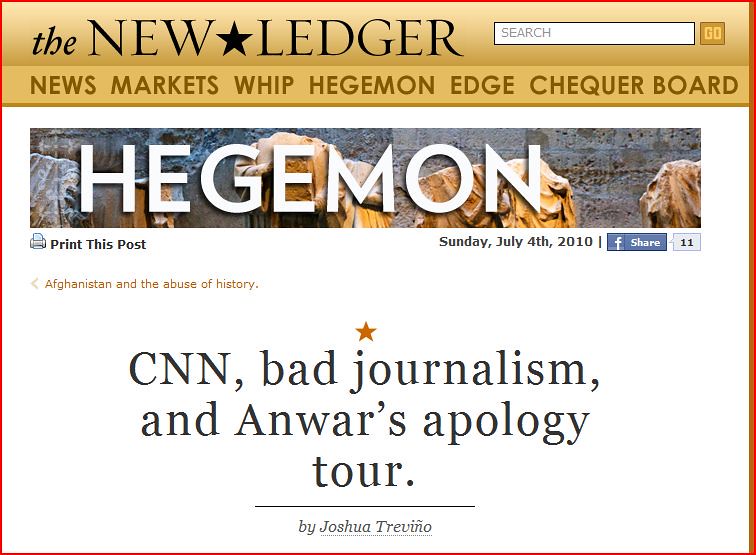This image appears to be a screenshot from a news website, featuring a detailed webpage layout. The top section is dominated by a thick, bronze-colored banner on the right and top edges, with a brown background. On the left side of the banner, "THE NEW LEDGER" is prominently displayed in all caps black letters, separated by a filled-in black star. To the right of this text, there is a white search bar. Below the banner, key navigation links read "NEWS, MARKETS, WHIP, HEGEMON, EDGE, CHECKERBOARD" against the brown background.

Beneath this banner, set against a white background, there's a large headline: "HEGEMON" in large white block letters with a rock and stone-patterned background. Below that, a black print icon and the text "Print This Post" are noted, with "Sunday, July 4th, 2010" and a Facebook share icon displaying '11' likes.

Further down the page, another prominent headline in the center reads, "CNN, Bad Journalism, and ANWR's Apology Tour," authored by Joshua Trevino, underlined by a thin black line. Additionally, toward the bottom centered text, there is a reference to previous content with a thin red back arrow and a note in small red font saying, "Afghanistan and the abuse of history."

The colors used throughout the webpage include brown, white, black, bronze, tan, gray, and red, contributing to the professional and detailed design typical of a news website interface.